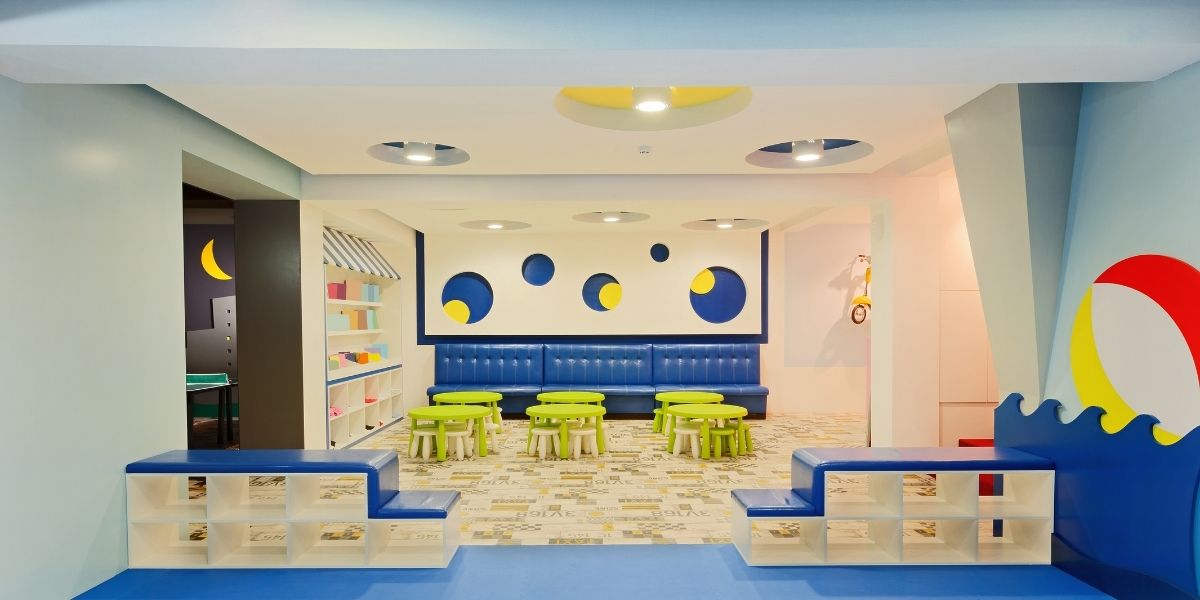The image depicts a vibrant and animated playroom inside a children's center. In the foreground, flanking both sides, are two sturdy shoe benches with cubby holes designed to store shoes, draped in a thick blue mat serving as a comfortable seating area. These are set on a blue floor. Moving into the background, the flooring transitions to brown and white tiles leading to six small lime green tables with white stools neatly tucked underneath them. Behind these tables, three blue booths are lined up next to each other, providing cozy seating against the wall. Above the booths, a large white painting features a pattern of overlapping blue and yellow circles, adding a playful touch to the decor. To the right, a wave motif is painted on the wall with a brightly colored beach ball above it, enhancing the whimsical atmosphere. On the left, more cubbies and shelves house various colored bags and art supplies, contributing to the organized yet lively environment. The ceiling lights, designed with blue and yellow circles, further illuminate the room, creating a cheerful and inviting space for children.